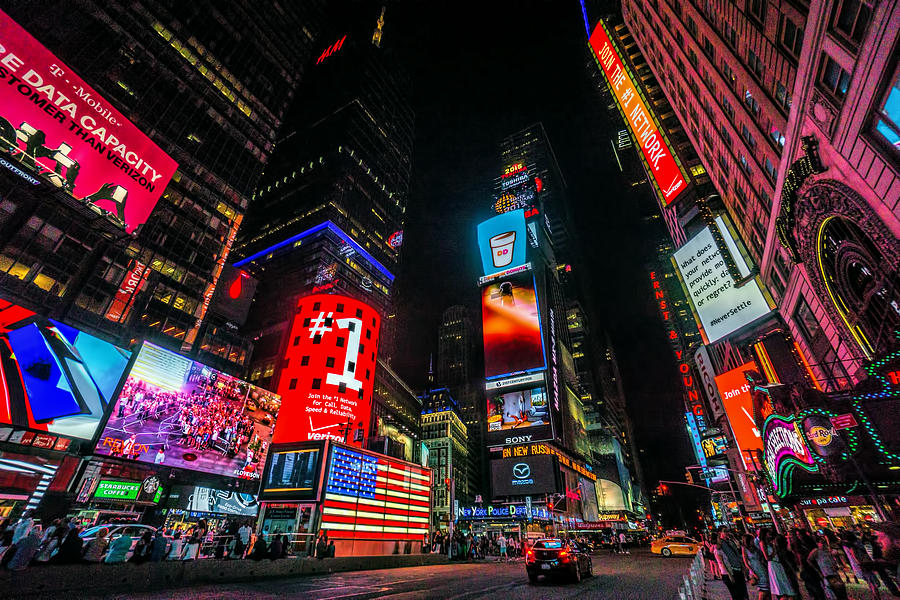This detailed photograph captures a vibrant night scene in Times Square, New York City, viewed from a very low angle almost at street level, with the camera tilted upwards, accentuating the dramatic height of the surrounding skyscrapers. The sky is devoid of any detail, pitch black, which contrasts sharply with the vividly illuminated buildings adorned with myriad neon signs and digital billboards. In the heart of this bustling square, an illuminated American flag shines brightly. Occupying prominent advertising spaces, brands such as T-Mobile, Verizon, Mazda, Sony, and Dunkin Donuts are visibly displayed in a variety of colorful neon lights. On the sides of the street, blurred images of numerous pedestrians are evident, though their features remain obscured due to the night-time setting and movement. A yellow taxi and a black vehicle can be seen driving on the illuminated streets. The rightward buildings are particularly striking with vertical neon signs and reflections of pink lighting from adjacent illuminated structures. The scene exudes an energetic and festive atmosphere, typical of one of the most iconic locations in New York City.